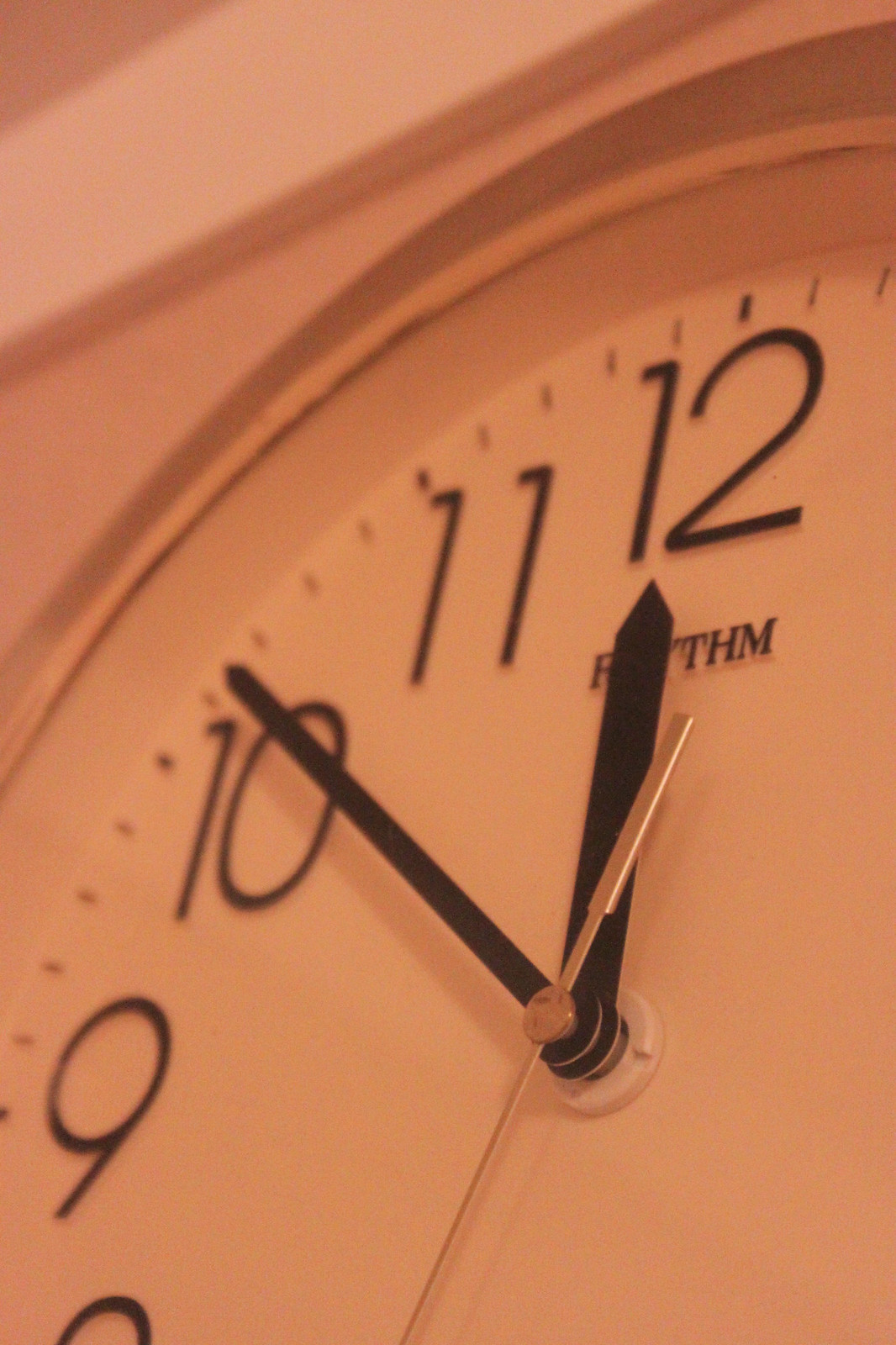This close-up photograph captures a modern clock face at a slight angle, highlighting the numbers 8 (partially), 9, 10, 11, and 12. The time displayed is approximately 9 minutes and 30 seconds to 12. The clock's hour and minute hands are black, while the metallic second hand is either gold or silver, reflecting different shades under the light. The clock face itself is a light beige or white color with black numbers and has a rim of very light brown beige. The brand name, likely "Rhythm," partially peeks from behind the clock hands, specifically below the 12. The upper left edge of the image includes part of the light beige wall and white ceiling border where the clock is mounted, further emphasizing the overall warmth of the scene's color palette.